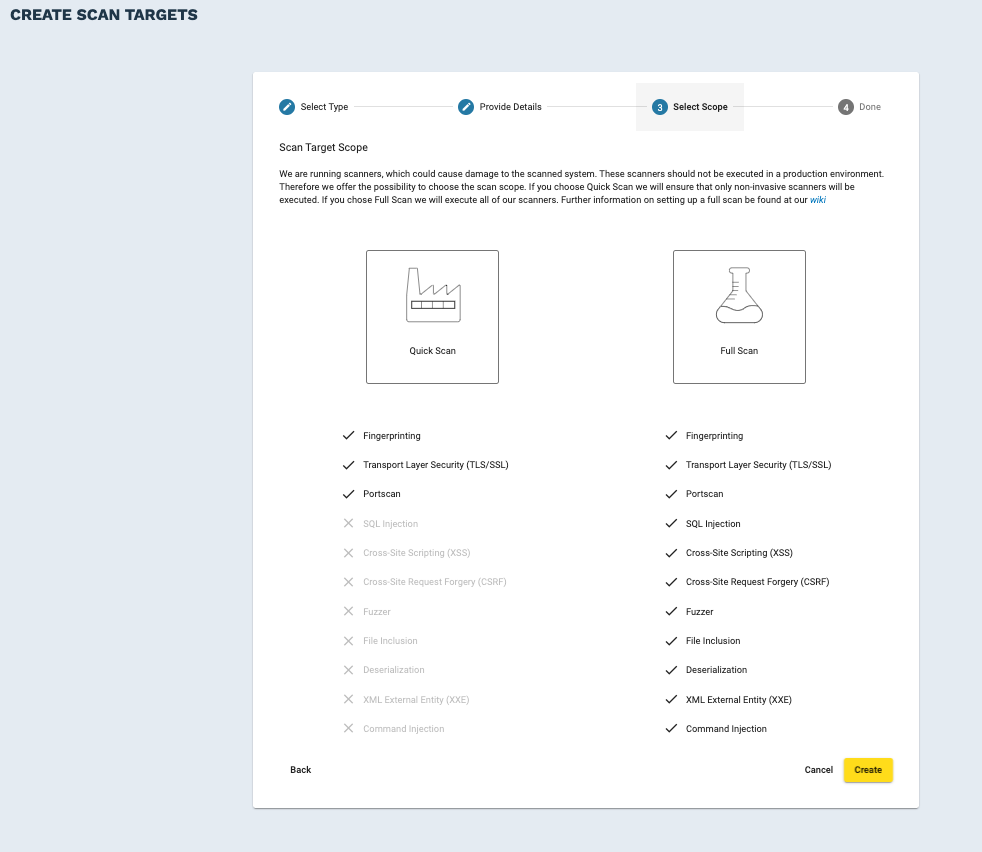The image is a screenshot capturing a webpage or an online science class program interface. At the top of the interface, in bold, all capital letters, the text "CREATE SCAN TARGETS" is prominently displayed in a dark blue font against a serene light or baby blue background. The main section of the screenshot features a white rectangular area that outlines a four-step process. These steps are sequentially labeled: "Select Type," "Provide Detail," "Select Scope," and "Done."

The first two steps, "Select Type" and "Provide Detail," are marked with a pencil icon, indicating that these have been completed by the user. The third step, "Select Scope," is highlighted with a gray box, signaling the current step in the process. The final step, "Done," awaits completion. Under the highlighted “Select Scope” step, the text "Scan Target Scope" appears along with a brief description.

Below this description, the user is presented with two scanning options: "Quick Scan" and "Full Scan," each represented by distinct icons. Accompanying these options is a checklist featuring various items marked with check marks and Xs, indicative of the selections or settings adjusted by the user thus far.